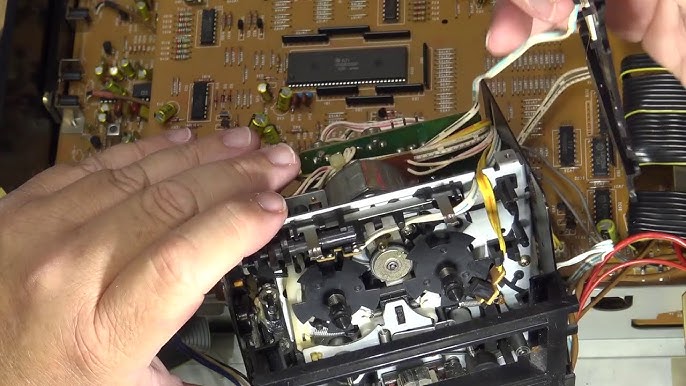This is a detailed, up-close, landscape-mode color photograph capturing the delicate process of repairing an intricate electrical device. The primary focus is on the fair-skinned hands of a person, particularly highlighting the left hand, which is holding a motorized component with an array of exposed wiring and mechanical parts, indicative of an interior motor stripped of its external casing. The right hand, partially visible, employs a black, tweezer-like tool to make precise adjustments within the small, complex areas of the device. Behind the hands, the detailed inner workings of a gold-colored motherboard with multiple soldered pieces, filaments, and diverse wiring can be observed. The setting appears to be a workspace with the device and motherboard resting on a white desk. The meticulous nature of the repair is emphasized by the presence of black and silver gears and various other intricate components, reflecting the complexity of this technical endeavor.